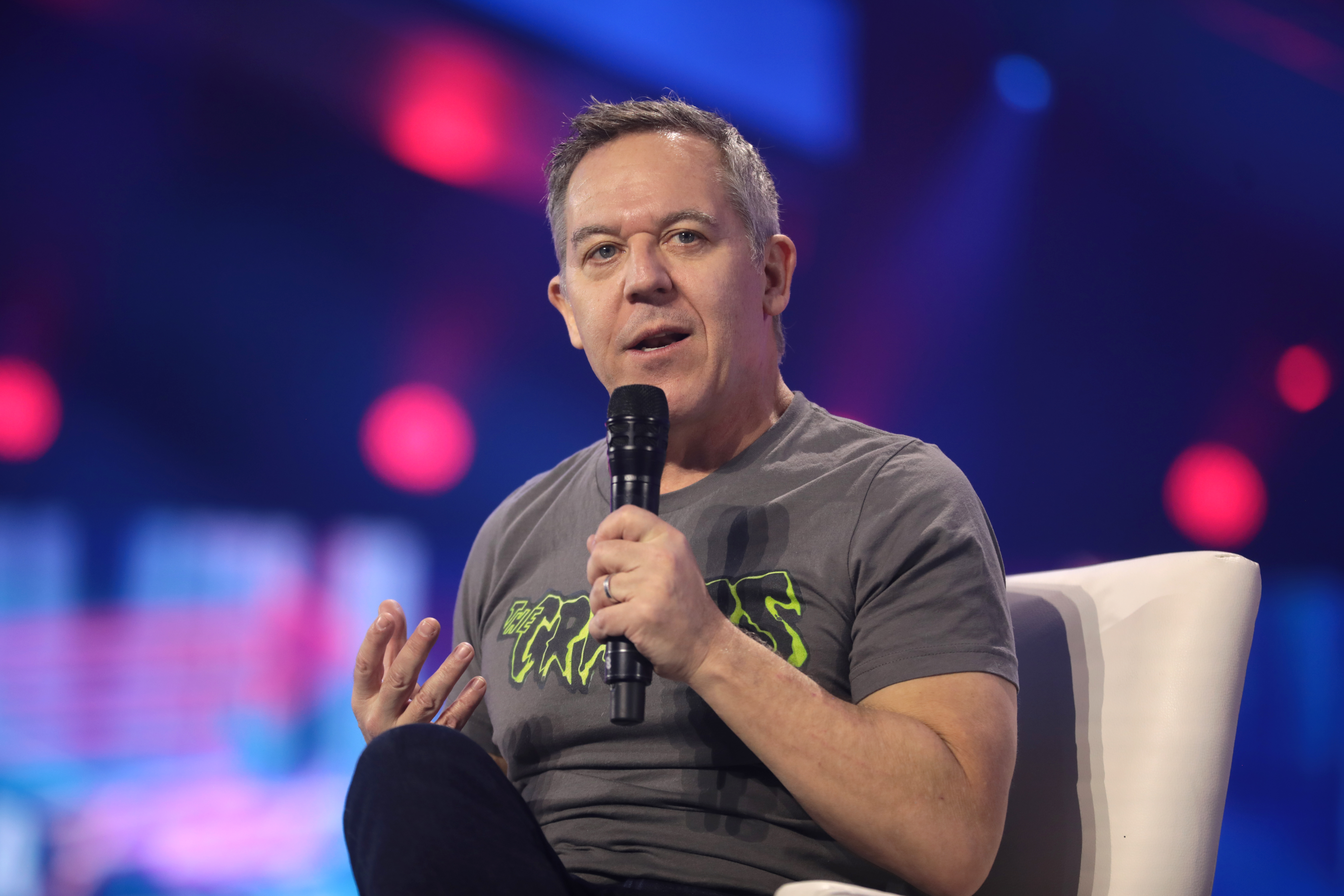This photograph showcases Greg Gutfeld, a Fox News host, seated in a white chair. With one leg crossed over the other, Greg holds a black microphone to his mouth with his right hand while gesturing animatedly with his left, suggesting he’s in the midst of delivering a humorous remark. He sports a gray t-shirt emblazoned with text reminiscent of superhero comic strips, partially obscured by his hand and microphone, revealing words outlined in green. Greg's short gray hair and blue eyes are clearly visible as he looks slightly upward. The background features a defocused, vibrant array of blue and red studio lights, adding a dynamic contrast that highlights his presence.